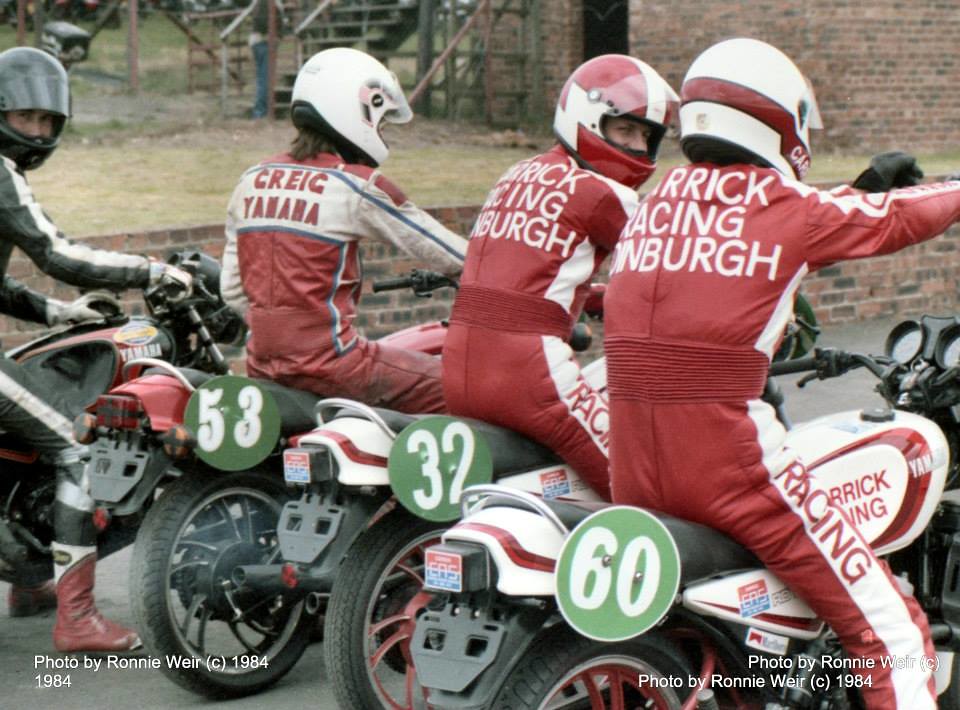The image captures four men poised on motorcycles, readying for a race on what appears to be an old, worn road. The three men on the right are donned in red and white racing suits with matching white helmets featuring red stripes. The farthest right rider's back displays lettering partially visible, likely reading "Merrick Racing Edinburgh." To his left, the next rider turns slightly towards the camera, his outfit similar in design and potentially bearing the same lettering. The third rider sports a red and white suit marked "Creek Yamaha" across the back and dons a plain white helmet. Meanwhile, the man on the far left stands out in a distinctive green suit with a matching green helmet. The motorcycles each have green circles with numbers on their rear fenders: 60, 32, and 53 from right to left. An old brick building with weathered wooden stairs and a grassy area with a person standing nearby appears to the left, suggesting a rustic setting. The photograph credits "Photo by Ronnie Weir, 1984" are noted in the bottom corners, confirming both the photographer and the year.